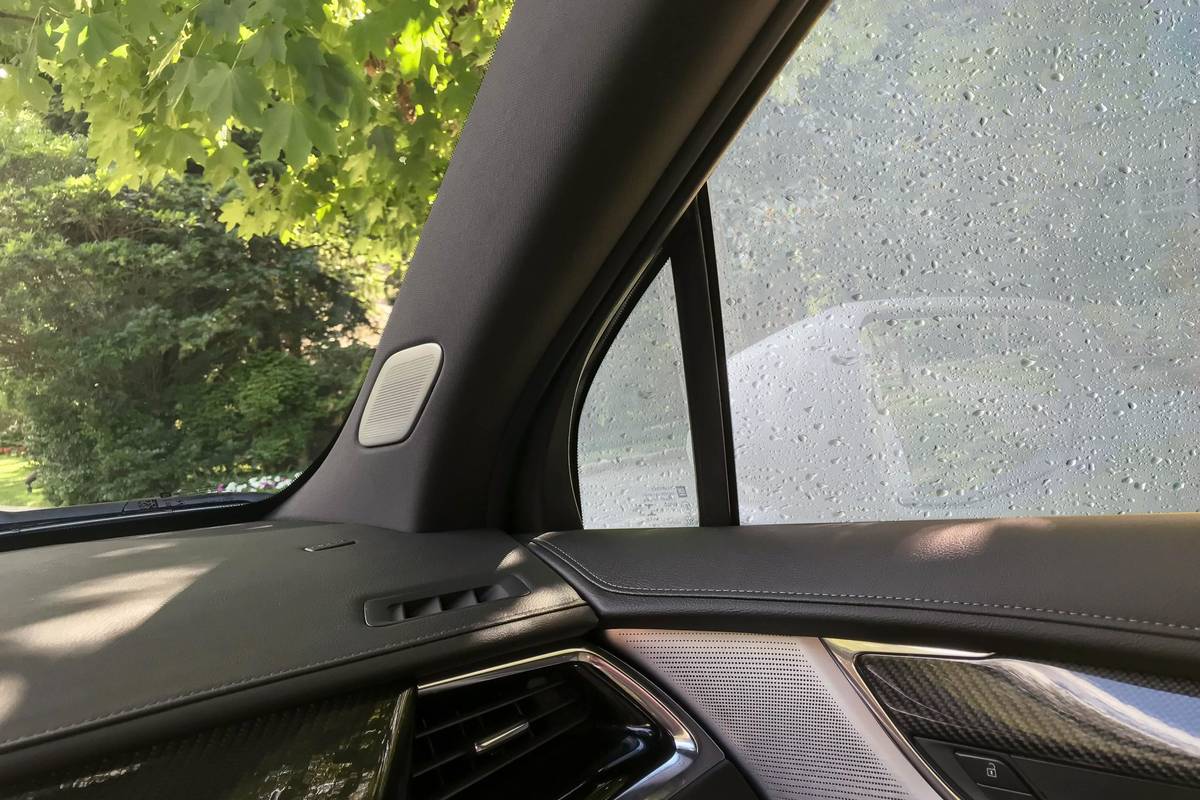This is a close-up color photograph taken from the front passenger seat of a car, offering a detailed view of its interior and the outside surroundings. The dashboard, primarily dark gray or blackish-gray, features clean lines and a visible air conditioning vent, speaker, and part of a carbon-patterned door handle. The passenger side window is heavily fogged and speckled with water droplets, making it difficult to see through; however, a faint outline of a white rearview mirror is barely visible. In contrast, the front windshield is clear, providing an unobstructed view of lush green foliage from nearby trees and bushes, with leaves potentially from an oak or grapevine hanging prominently. The curved windshields and the frosted appearance of the side window add depth to the cozy and damp atmosphere inside the vehicle.